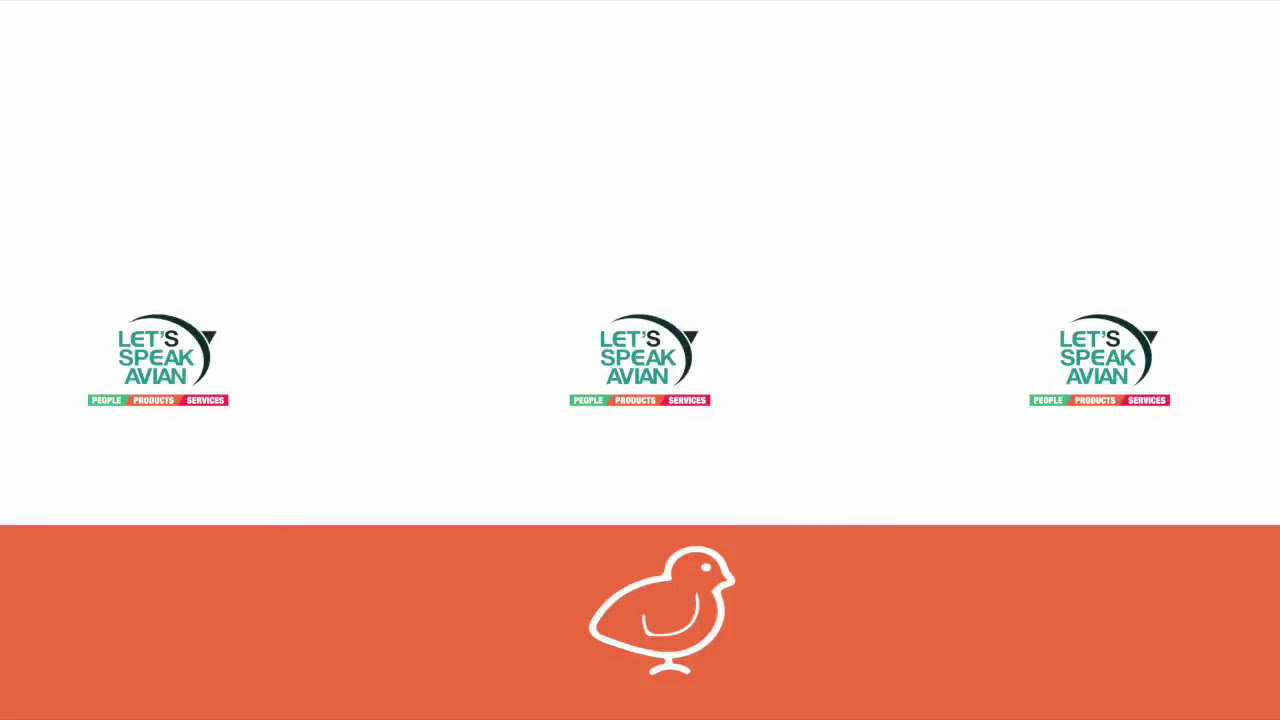The image appears to be a digital poster with a primarily white background. The lower portion of the poster features an orange rectangular strip that spans the width of the image. On this strip, there is a detailed line drawing in white of a baby bird in profile, facing right, with its feet visible. Above the orange strip are three identical logos, each comprising a black triangle-like swoosh followed by the text "Let's Speak Avian." Notably, the 'S' in 'Let's' is black, while the rest of the text is green. Below each logo, the slogans "People," "Products," and "Services" are displayed in distinct color blocks: blue for 'People,' orange for 'Products,' and red for 'Services.' The repetition of the logo and text adds to the overall symmetry and structure of the design, suggesting a digital creation or printout for a website or promotional material.